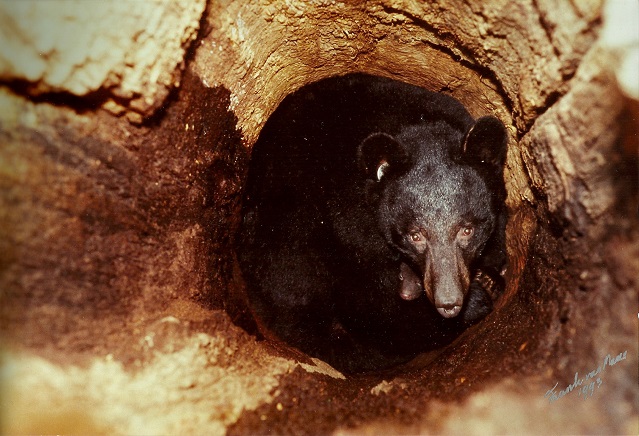The photograph captures a poignant moment of a large bear, likely a black bear, nestled inside a log den and gazing towards the camera. The scene exudes an earthy palette with various shades of brown, capturing the surrounding bark and the bear's fur. The bear is accompanied by its cub, which is nestled beneath its chin, adding a tender element to the composition.

The bear's long nose and distinct, rounded brown ears are prominently visible, framing its sad, brown eyes that suggest it might be in distress. Light filtering into the den casts a series of shadows and light patches across the bark and the bear's fur, highlighting individual strands and adding texture to the image. 

An ear tag on the bear hints that it may be part of a tracking study, underscoring the significance of this intimate wildlife moment. The photograph appears to be taken either from above or at an angle, providing a clear view into this secluded bear family. The image's dated watermark, likely from 1993, adds an element of archival value to this well-lit and detailed snapshot of bear behavior in the wild.